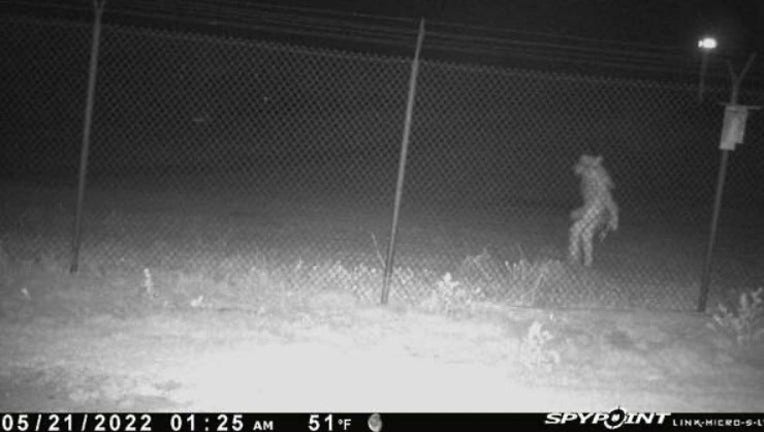The image, taken by a Spy Point security camera, displays date and time data of 05/21/2022 at 01:25 AM with a temperature reading of 51 degrees Fahrenheit. Captured in a dimly lit, black-and-white night setting, the central focus is a chain link fence topped with double-pronged Y-shaped barbed wire. Behind and to the right of the fence, an upright figure can be seen. The figure appears to have big ears, a short snout, and a long, hairy mane, giving it an eerie, almost man-shaped yet distinctly odd appearance, enhancing the mysterious atmosphere of the scene. The textual information on the image is primarily white, contrasting against the dark background, adding to the overall sense of intrigue and ambiguity.